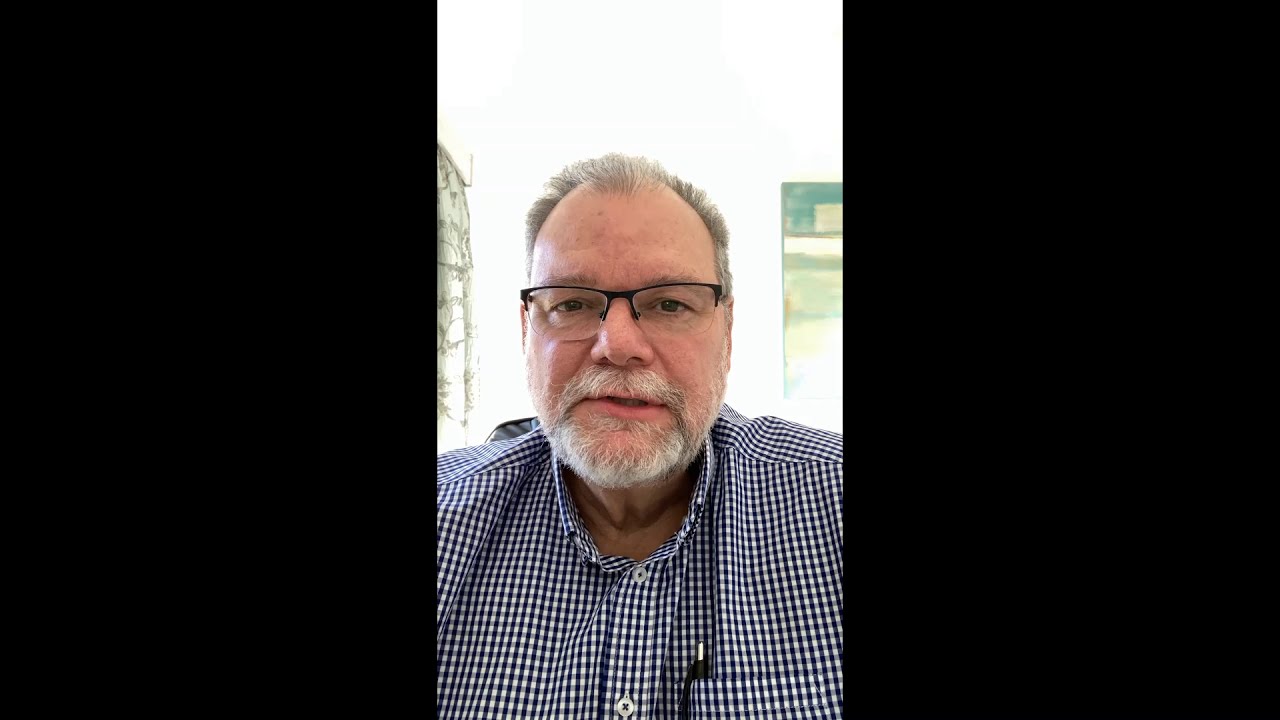An elderly white man with a receding hairline and a mixture of gray and black hair stares straight forward. He has a full beard and mustache, predominantly gray with some black strands, and brown eyes behind black half-rim glasses. His mouth is partially open as if speaking mid-sentence. He is wearing a blue and white checkered button-up shirt with a black pen sticking out of the pocket. The background features a bright, blurred white wall with a teal-to-yellow gradient picture hanging on the right side and a window with brown trim on the left. The left and right thirds of the image are framed by black columns.